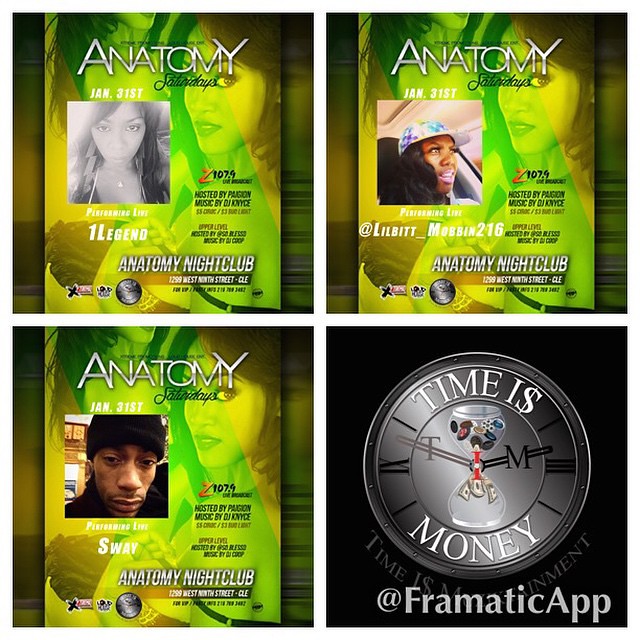The image is divided into four quadrants, resembling a window with white stripes crossing vertically and horizontally. The background of three quadrants (top left, top right, and bottom left) features a hot green and yellow color scheme with a woman's silhouette. These three sections advertise "Anatomy Saturdays" at the Anatomy Nightclub with a Z107.9 radio station promotion. The details on each are slightly different:

- The top left quadrant showcases a black and white picture of a woman with long black hair, labeled "One Legend," dated January 31st.
- The top right quadrant features a woman wearing a rainbow-colored baseball cap, identified as "Lil' Bit" and mentions "Morbin 216."
- The bottom left quadrant displays a man with a black knit cap, named "Sway."

The bottom right quadrant diverges from the others, having a logo with the phrase "Time is Money" and mentioning the "Chromatic App."